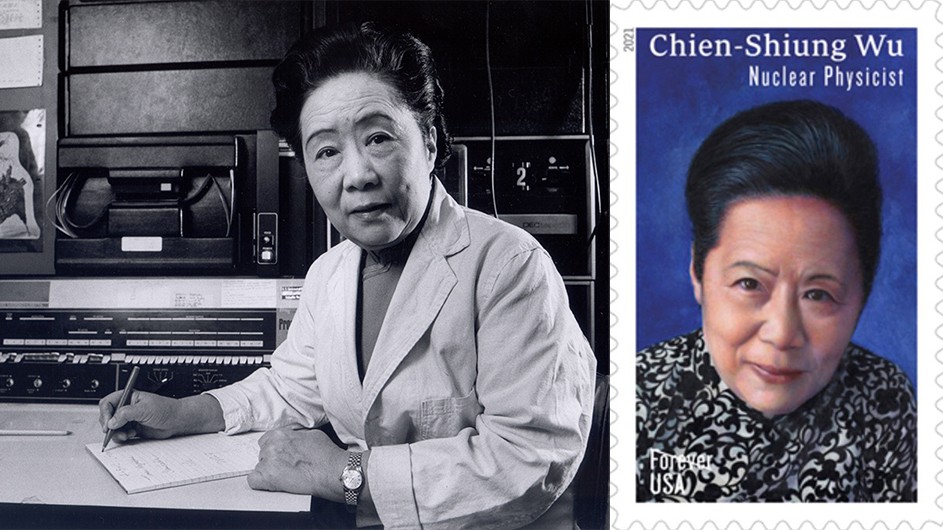The composite image features two representations of a renowned nuclear physicist named Chien-Shiung Wu. On the left is an older black-and-white photograph, likely from the 1970s, capturing Wu in her laboratory. In the image, she appears to be in her 50s or 60s, dressed in a lab coat. Wu is seated at a table with a lined tablet in front of her and a pen in her right hand. She is looking directly at the camera with a neutral expression, her left hand resting on the table, displaying a wristwatch. Her hair is neatly pulled back from her face.

On the right side is a contemporary color image of a U.S. Forever postage stamp issued in 2021. The stamp features a photograph of Wu against a dark blue background, showcasing her with a pleased expression. She is wearing a black and white print top. The stamp includes the text "Chien-Shiung Wu, Nuclear Physicist" at the top, celebrating her significant contributions to the field of nuclear physics.